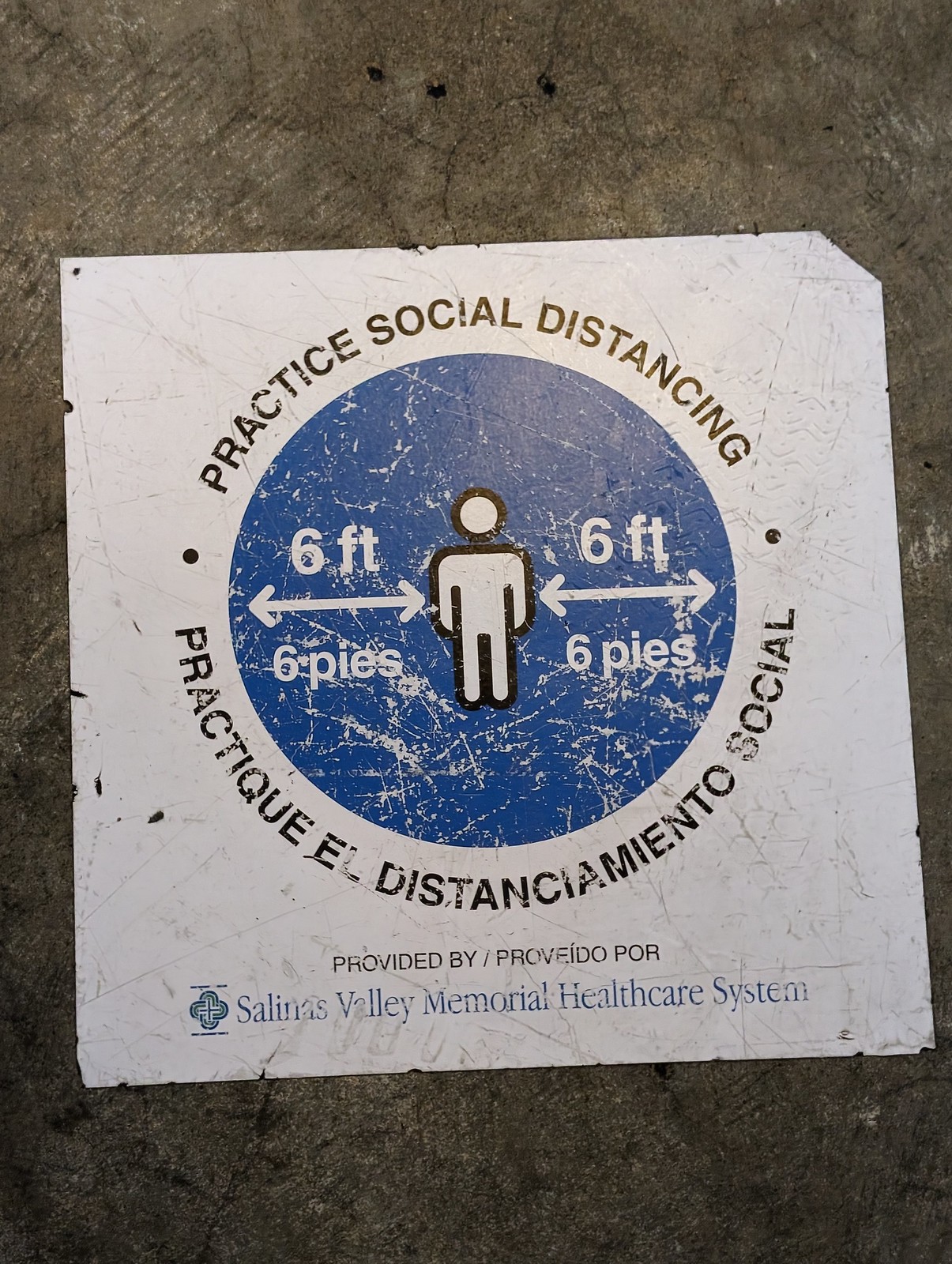The image depicts a poster situated either on a wall or the ground, against a cement surface marked by three holes at its top. The poster itself is white and has multiple holes, suggesting it could be made of either paper or cardboard. Dominating the center of the poster is a large blue circle. Within this circle, the text "Six Feet" is displayed, accompanied by an icon of a person flanked by arrows pointing left and right to indicate the six-foot distance. Surrounding the circle is the phrase "Practice Social Distancing." Below this primary message, there's additional text in another language, and at the very bottom of the poster, it reads "Provided by Salinas Valley Memorial Healthcare System."